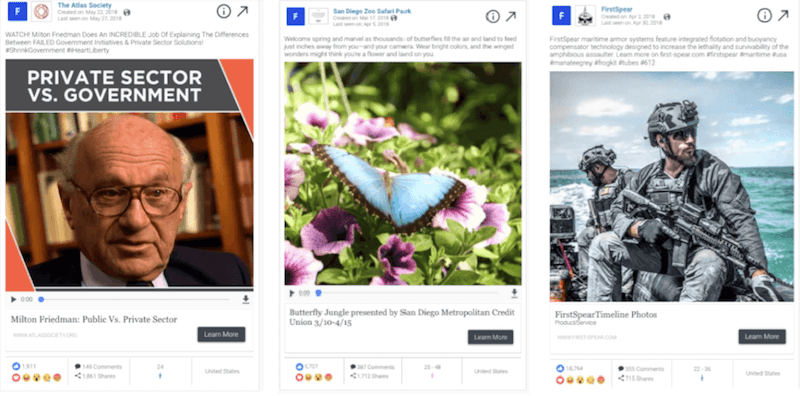The blurry image contains three distinct visual elements, each featuring a brief news story or audio feature. Despite the lack of clarity, some details can be discerned:

1. **Left Section:**
    - **Image:** An elderly individual, likely in their 70s or 80s, looking directly at the camera.
    - **Headline:** "Private Sector vs Government."
    - **Subheadline:** "Milton Friedman: Public vs Private Sector."
    - **Button:** A clickable button labeled "Learn More."
    - **Social Stats:** Displays various social interaction options such as emojis, share functionality, view count, and the publication location, noted as the United States.

2. **Middle Section:**
    - **Image:** A blue butterfly with black-edged wings perched on purple petunias.
    - **Headline:** "Butterfly Jungle."
    - **Sponsor:** "Presented by San Diego Metropolitan Credit Union."
    - **Date:** "3/10/2015."
    - **Button:** A clickable button labeled "Learn More."
    - **Social Stats:** Includes emojis, sharing options, view count, and the publication location, noted as the United States.

3. **Right Section:**
    - **Image:** Two soldiers, possibly from the Navy, are seen on a boat navigating in open waters.
    - **Headline:** "First Spear Timeline Photos."
    - **Button:** A clickable button labeled "Learn More."
    - **Social Stats:** Features emojis, share options, view count, and the publication location, noted as the United States.

While the images are blurry and some text is difficult to read, the layout provides an overview of various topics ranging from economic discussions and nature exhibits to military activities. Each section provides user engagement options and is predominantly published in the United States.